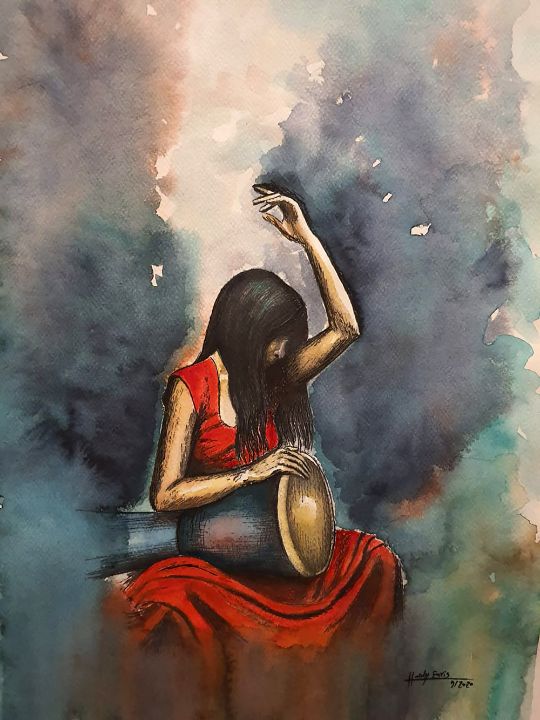The painting depicts a woman seated at the center of a rectangular canvas, with the left and right sides twice as long as the top and bottom. She is wearing a short-sleeve red dress with a low neckline and has long black hair that obscures most of her face, leaving only her nose and part of her mouth visible. The woman is engaged in playing a black drum with a white drum head, which rests on her right knee. Her right arm drapes over the drum while her left arm is lifted, poised to strike. The background is predominantly blue, but it features a white streak rising behind her, and there are diverse splotches of other colors such as greens, browns, teals, purples, pinks, and peach, adding layers of complexity. In the bottom right corner of the painting, the artist's signature is visible in black ink. The scene conjures an image of calm amidst chaos, as if she is in an environment filled with smoke and debris, suggesting the painting might symbolize endurance and expression in the face of adversity.